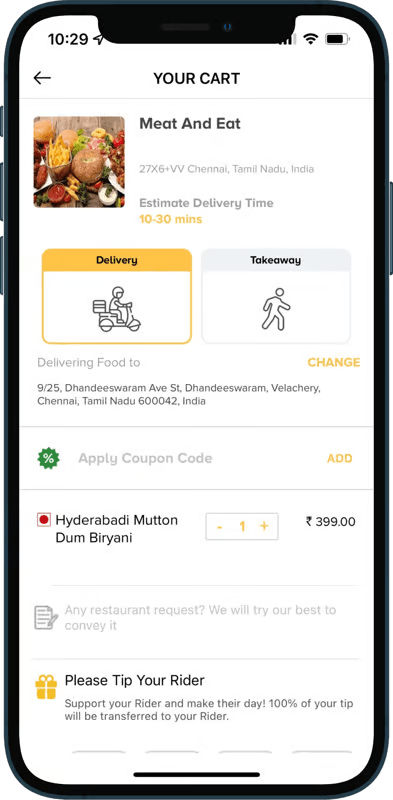The image depicts a smartphone screen, held against a black background. The smartphone displays an interface related to a food delivery service named "Tompas 1029". At the top, the phone shows a full Wi-Fi signal and an almost fully charged battery icon. The visible interface features a left arrow indicating a back navigation option.

Prominently, there's a card showing an image of various meats and fries, likely representing one of the menu items. The card also displays the text "Meat and Eat".

Below, additional details include "27X6 plus Phoebe", "Channel, Tamil Nadu, India", and an estimated delivery time of "10 to 30 minutes". The estimated delivery time appears twice. Yellow squares emphasize the delivery information, which is accompanied by an image of a man on a scooter, evidently the delivery person.

The address for delivery has been updated to "925 Avenue Street, Chennai, Tamil Nadu, India".